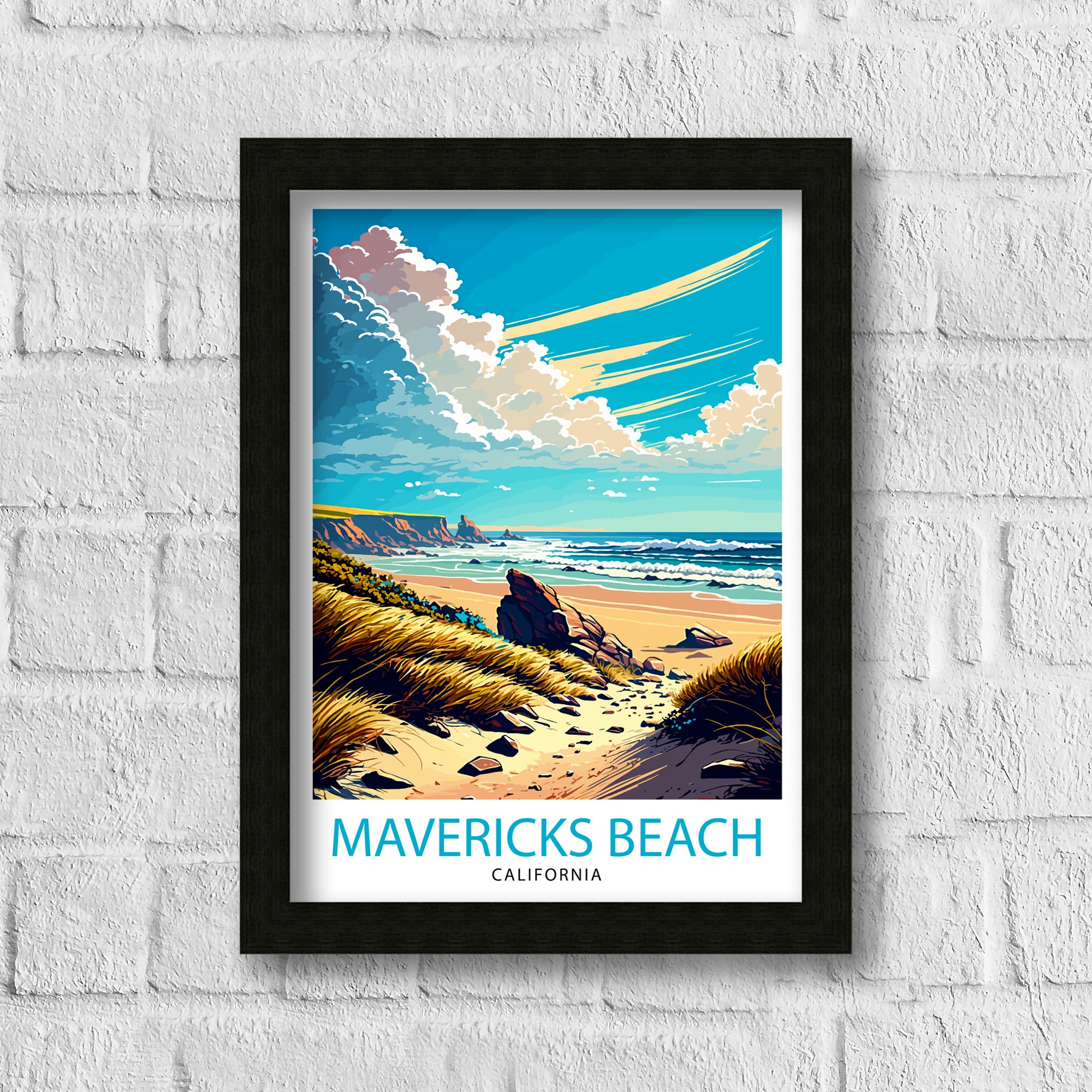This image showcases a prominent framed poster mounted on a white-painted brick wall. The black wooden frame encases a detailed graphic artwork titled "Maverick's Beach" in bold, light blue capital letters with "California" written below in smaller black font. The artwork vividly depicts a scenic beach setting featuring a sandy path flanked by tall grass and sand dunes, leading down to a tranquil beach. In the background, waves crash against scattered rocks and cliffs, all beneath a sky filled with both serene clouds and stormier patches, suggesting an impending storm. The overall composition captures the rugged beauty and dynamic atmosphere of Maverick's Beach, California.